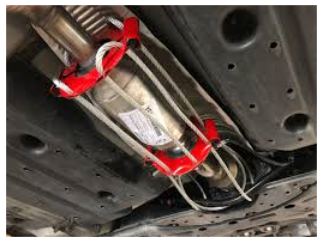The image depicts the underside of a car, focusing prominently on the catalytic converter. The entire undercarriage is painted black, while the catalytic converter itself is a shiny, cylindrical, silver component positioned centrally. This catalytic converter is surrounded by a contraption that appears to be a makeshift security measure—a clear plastic tube encasing a metal chain, akin to a bike lock, wound around the converter to deter theft. Enhancing this DIY anti-theft device are red brackets positioned both in front of and behind the catalytic converter. Additionally, there's an element of red ribbon attached to this system, seemingly helping secure the entire assembly in place. The clarity of the image and the well-lit setting make all these components distinctly visible.